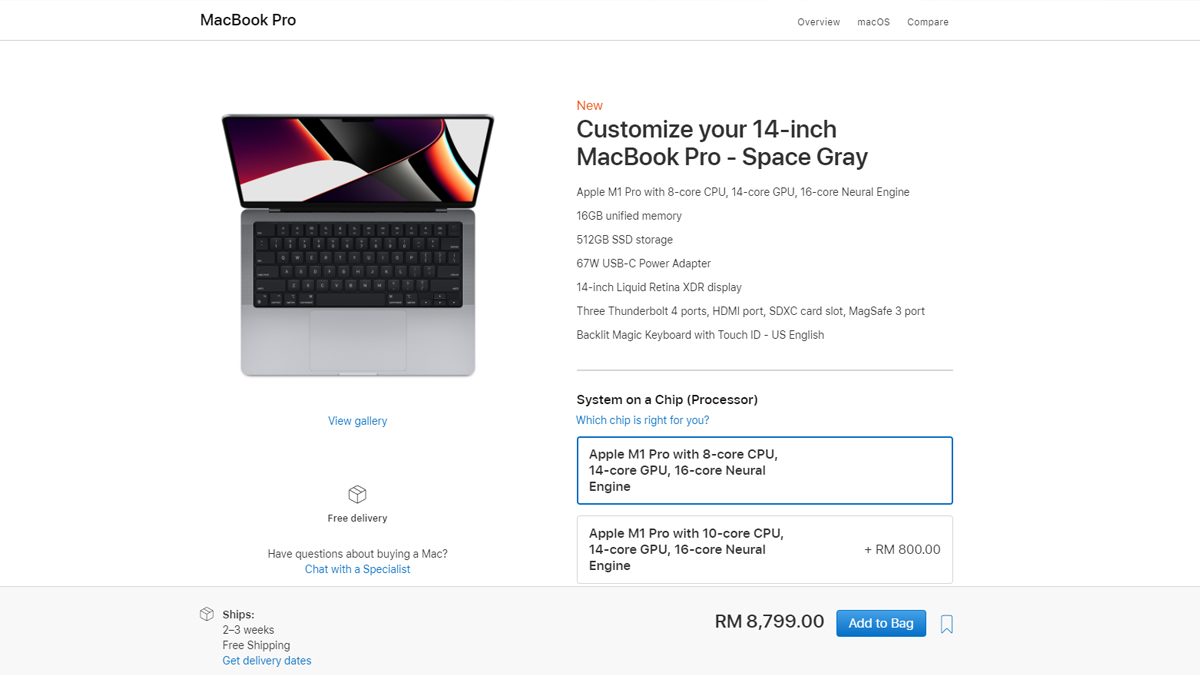This image appears to be a screenshot from the official MacBook Pro website, featuring a prominently displayed MacBook Pro on the left side of the page. The MacBook Pro showcased in the image is sleek and silver, with a striking black keyboard. 

Below the image, there is a blue link labeled "View Gallery," inviting users to explore more photos of the MacBook Pro. Just beneath this link, there is a small box icon with text stating "Free Delivery." 

Further down, there is a section with a question about purchasing inquiries: "Have questions about buying a Mac?" followed by a "Chat with a Specialist" prompt in blue text, urging users to seek assistance.

At the top right corner, a red tag reads "New," followed by the headline in bold black text: "Customize your 14-inch MacBook Pro – Space Gray." This section provides detailed specifications including 16GB of unified memory, information about storage options, power adapter details, display features, and highlights on the three Thunderbolt 4 ports.

Continuing down the page, there are details about the system on a chip, including processor options, and a section helping users decide which chip is best for their needs. The selected option here appears to be a chip with a 14-core GPU and a 16-core Neural Engine, indicative of a powerful and high-performance device.